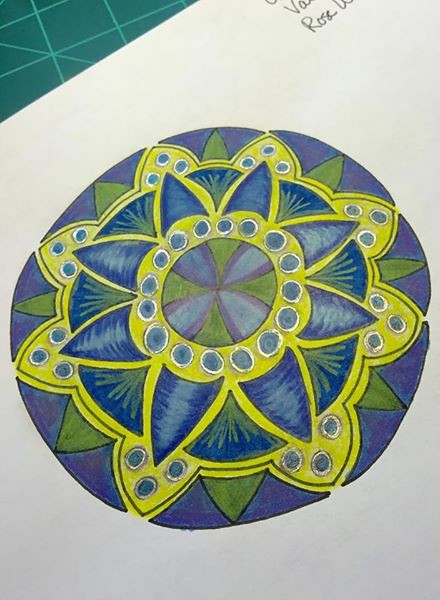This detailed and vibrant photograph showcases a meticulously crafted mandala drawing, likely created on a white sheet of sketchbook or printer paper. The artwork, which could possibly be a colored page from a coloring book, features intricate patterns and a harmonious blend of colors. The mandala is primarily shaded using colored pencils or pastels, evidencing a waxy texture.

The color palette starts with a light green, almost yellow, base, adorned with blue dots on each petal on the outer rim. Progressing inward, the layers reveal a gradient of darker and lighter blues, culminating in a center imbued with rich purples. The outermost edge of the mandala also incorporates shades of purple, adding to the visual depth and symmetry.

In the upper right corner, there is a marking that might be the artist's signature, lending a personal touch to the piece. The entire drawing is set against a green cutting mat with light green gridlines, providing a structured background that complements and highlights the details of the mandala.